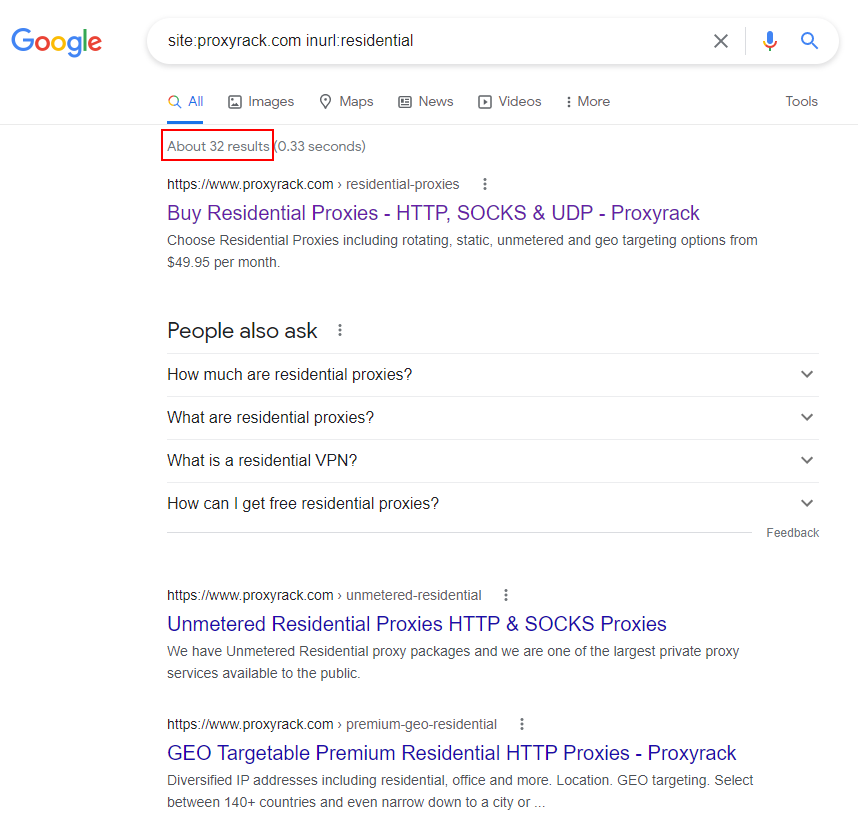The image depicts a Google search results page. At the top left corner, the Google logo is visible, displaying the brand name in blue, red, yellow, and green letters. Below the logo, the search bar contains the query "site:proxyrack.com residential." Beneath the search bar, various navigation options are listed, including "All," "Images," "Maps," "News," "Videos," "More," and "Tools." The page indicates approximately 32 search results, a section that is highlighted with a red box likely added through editing.

The first search result listed is from proxyrack.com, providing information about purchasing residential proxies. It states: "Proxy Rack: Buy Residential Proxies - HTTP, SOCKS, and UDP. Proxy Rack offers residential proxies, including rotating, static, unmetered, and geo-targeting options for $49.95 per month."

Further down, a "People also ask" section lists frequently asked questions such as "How much are residential proxies?", "What are residential proxies?", "What is a residential VPN?", and "How can I get free residential proxies?"

The second search result reiterates Proxy Rack's services: "Proxy Rack: Unmetered Residential Proxy - HTTP and SOCKS proxies. We have unmetered residential proxy packages. We're one of the largest private proxy services available to the public."